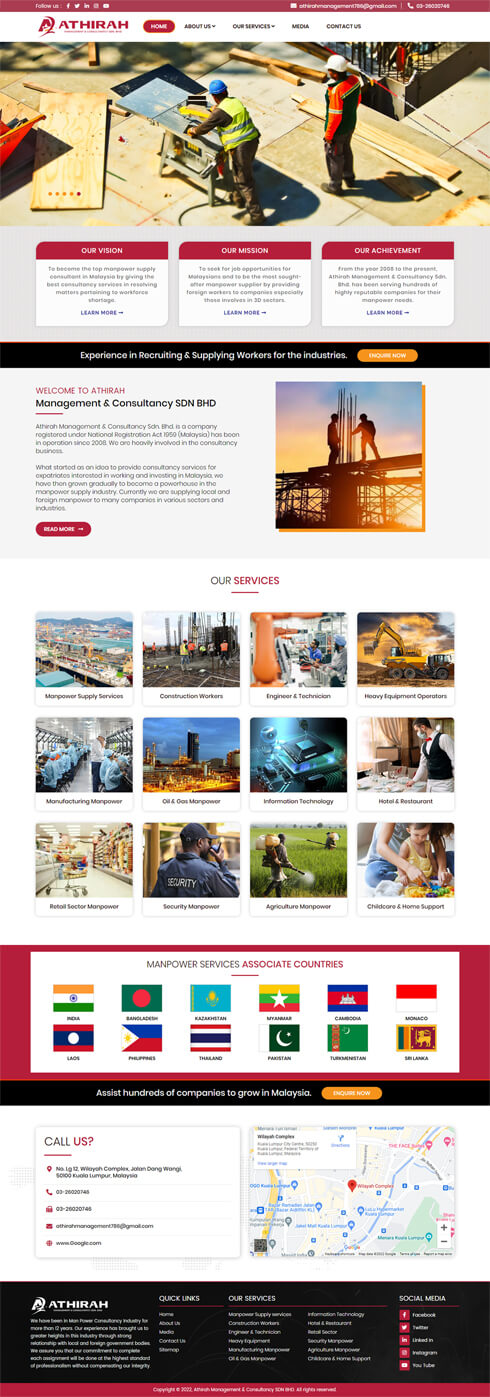The image shows a website dedicated to a construction-related company, though zooming in reveals significant blurriness, obscuring finer details. At the top of the page, there's a red banner labeled "Follow Us," featuring recognizable social media icons for Facebook, Twitter, LinkedIn, YouTube, and possibly Instagram, indicated by a camera icon. Also present is the Gmail logo.

The background below this section turns white, with the company's name displayed prominently in red: "ATHIRA." This is accompanied by navigation buttons in a red oval, including "Home" in white text. Other navigation options such as "About," "Our Services," "Media," and "Contact Us" are listed in black. 

Further down, another section has a heading in red text reading "Our Vision," partially legible as aiming to become a top manpower management or supply consultant. "Our Mission" follows, mentioning the goal of seeking job opportunities, though much of the text is unreadable.

Achievements from 2008 to the present are briefly mentioned but are largely unclear. The background transitions to black, with a white text overlay stating the company's extensive experience in recruiting and supplying workers for various industries.

Lastly, an orange section with white text urges visitors to "Inquire Now," and another segment highlights "Manpower Services" in red. This area identifies their associate countries, including India, Bangladesh, Cambodia, Sri Lanka, Pakistan, Thailand, the Philippines, and Laos.